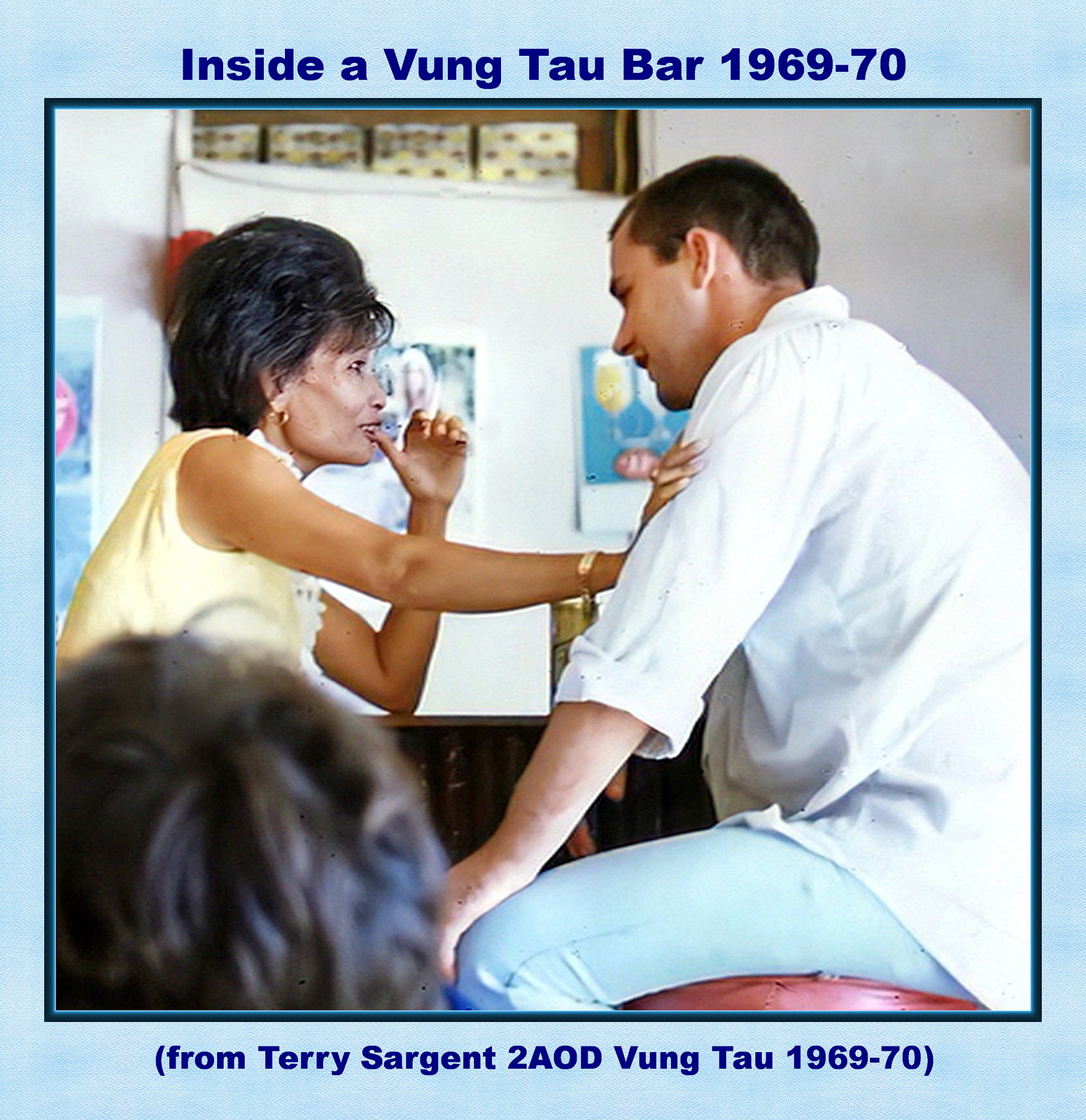The image is a color photograph taken indoors, framed by a light blue outer border with a dark blue inner border and a black drop shadow. At the top of the border, blue text reads "Inside of Vung Tau Bar, 1969-70," and at the bottom, it says "From Terry Sargent to AOD, Vung Tau, 1969-70."

In the photograph, a Caucasian man and an Asian woman are seated facing each other. The man, on the right side of the image, is wearing a long-sleeve white button-up shirt with the sleeves rolled up and light blue jeans. He has short dark hair and is smiling at the woman, with his left hand resting on his knee.

The woman, seated on the left side, is wearing a sleeveless yellow top and has dark, voluminous hair. She has her right arm extended, resting her hand on the man’s left bicep, while her left hand is near her mouth. She is gazing directly at the man.

Behind them, the background features a wall adorned with canvases or posters, possibly including pictures of beer glasses. In the lower left corner of the photograph, the back of a dark-haired person's head is partially visible.